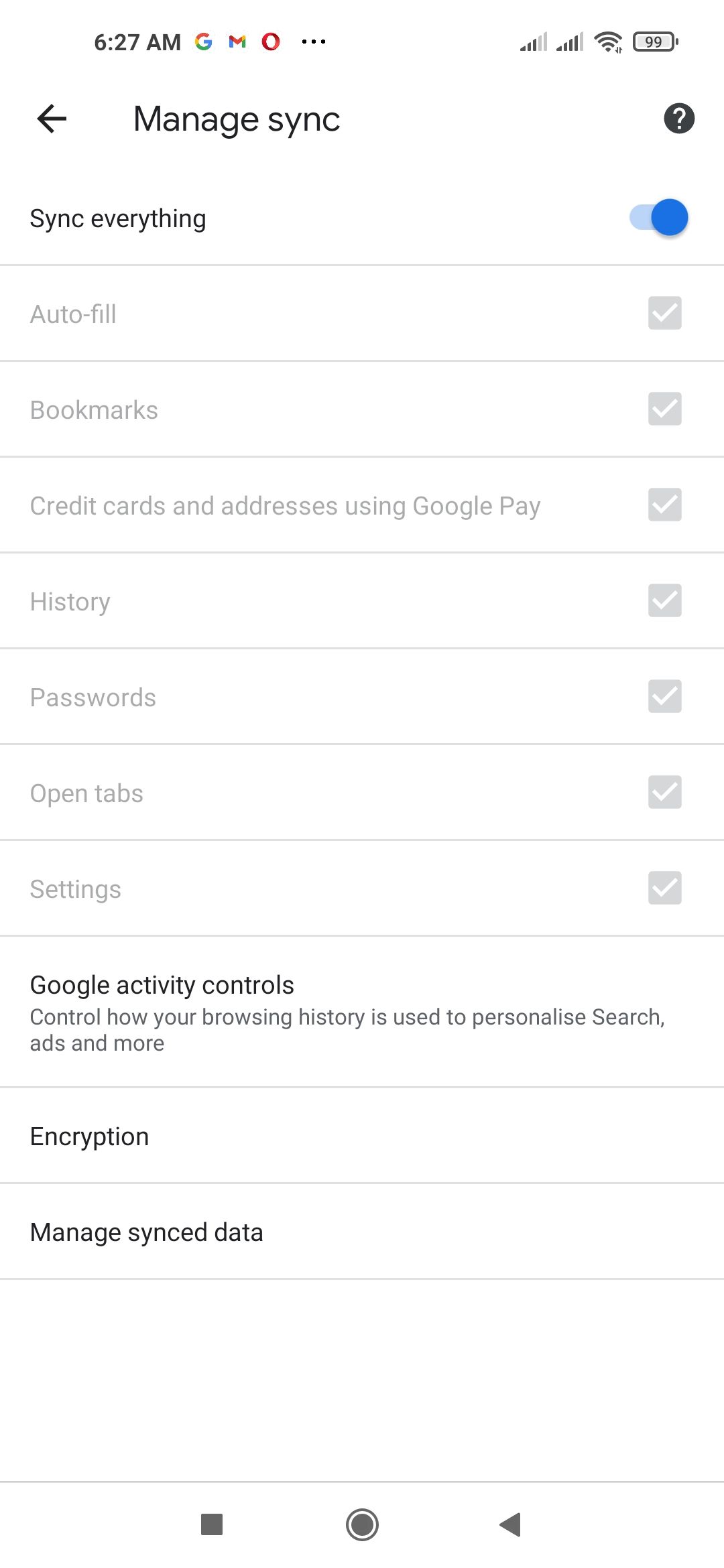This image is a detailed screenshot of the "Manage Sync" settings page for a Google account on a mobile device. At the top of the interface, a back arrow icon appears next to the text "Manage Sync," and a question mark icon on the right offers help or additional information. The status bar shows the current time as 6:27 AM, with a battery level of 99% and network icons indicating connectivity.

Immediately below the header is a prominent switch labeled "Sync Everything," which is turned on and highlighted in blue, indicating that all sync options are enabled. Beneath this switch, various sync options are listed, each accompanied by a checkbox indicating they are enabled. These options include syncing for Autofill, Bookmarks, Credit Card history, and Open Tab settings.

Further down, the screen provides access to "Google Activity Controls," with a brief description that explains how to manage browsing history, personalized search ads, and other settings. Additional options for encryption and managing synced data are also available.

The overall design of the page is simple and clean, featuring a white background with black text. The layout and style are consistent with other Google products, making it familiar and user-friendly.